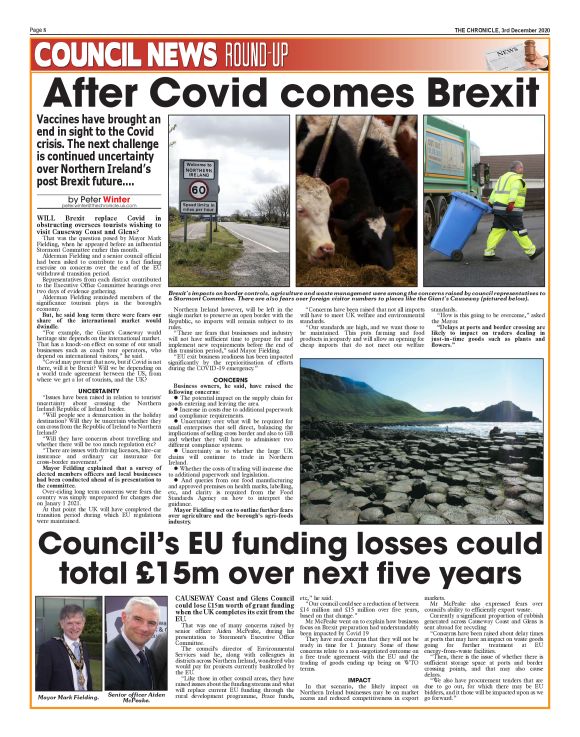This image shows a newspaper entitled "Council News Roundup." The prominent message is, "After COVID Comes Brexit," highlighting the transition from the pandemic's conclusion, attributed to successful vaccine rollouts, to ongoing uncertainties concerning Northern Ireland's post-Brexit future. A lengthy article explores this issue. The newspaper also includes several images: one of a roadway with a speed limit of 60, another of cows eating hay, and a third of a sanitation worker pulling a blue barrel, which indicates recycling, though its significance in Ireland is unclear. Another headline reads, "Council's EU Funding Losses Could Total $15 Million Over the Next Five Years," accompanied by an article on the topic. However, the print of these stories is extremely small, and the website hosting the newspaper image does not allow the text to be enlarged for better readability; increasing the image size only magnifies the instructions, not the content itself.